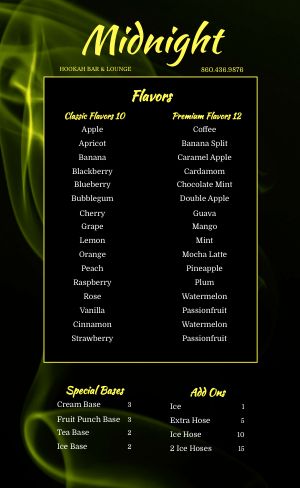This image appears to be a menu sign for a hookah bar and lounge, set against a primarily black background with green and yellow smokey effects in the top left corner. At the top center, the text "Midnight Hookah Bar and Lounge" is prominently displayed in yellow, along with the phone number 880-438-9578. Below this, the menu is presented within a black rectangle bordered by the same greenish-yellow color. The menu is divided into sections: "Flavors," "Special Bases," and "Add-Ons."

Under "Flavors," there are two categories:
- **Classic Flavors (10):** Apple, Apricot, Banana, Blackberry, Blueberry, Bubblegum, Cherry, Grape, Lemon, Orange, Peach, Raspberry, Rose, Vanilla, Cinnamon, Strawberry.
- **Premium Flavors (12):** Coffee, Banana Split, Caramel Apple, Cardamom, Chocolate Mint, Double Apple, Guava, Mango, Mint, Mocha Latte, Pineapple, Plum, Watermelon, Passion Fruit (with Watermelon and Passion Fruit repeated twice).

At the menu's bottom center, the sections for "Special Bases" and "Add-Ons" are listed:
- **Special Bases:** Cream Base 3, Fruit Punch Base 3, Tea Base 2, Ice Base 2.
- **Add-Ons:** Ice 1, Extra Hose 5, Ice Hose 10, 2 Ice Hoses 15.